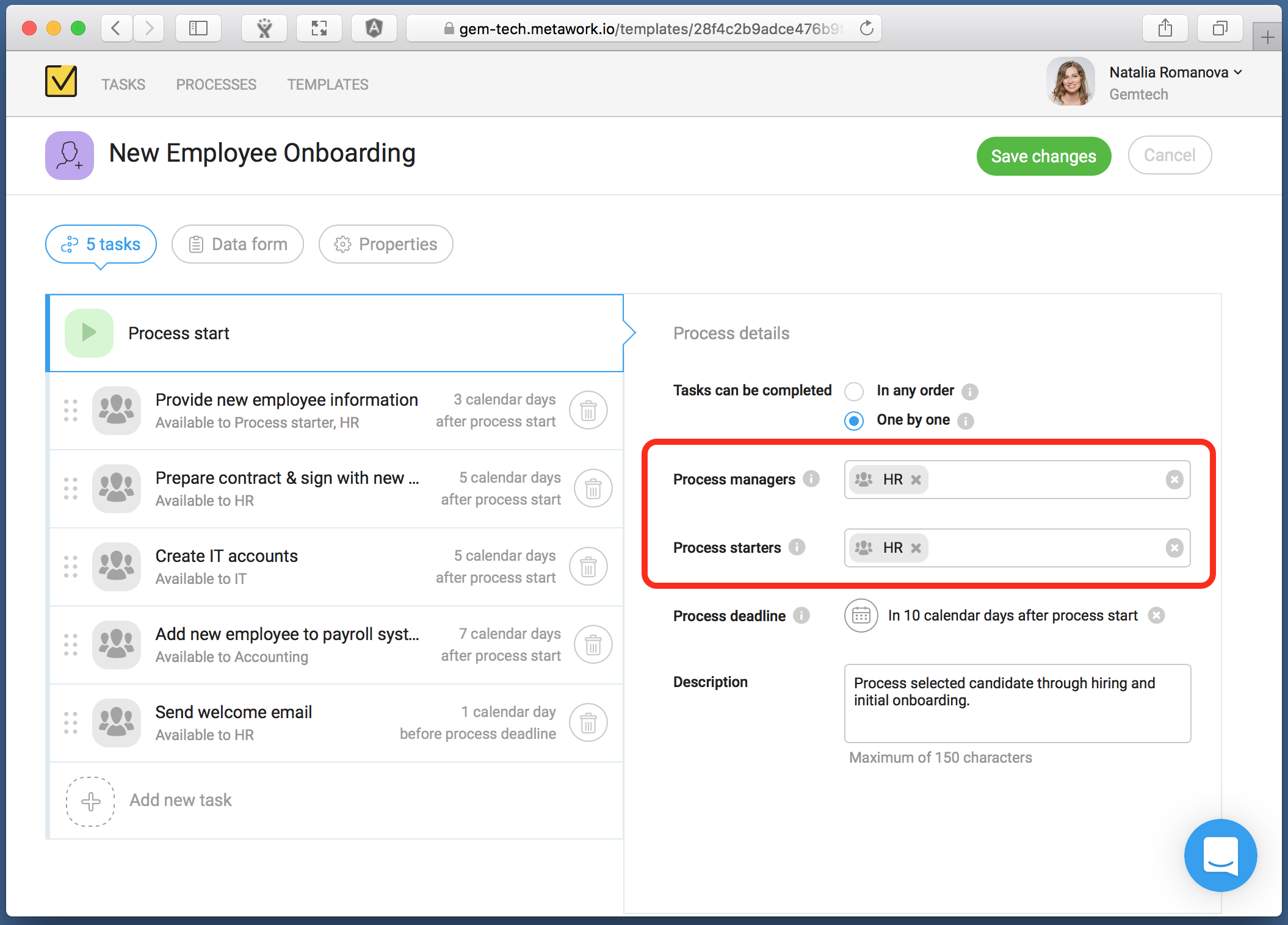**Screenshot of New Employee Onboarding Screen**

The screenshot showcases a new employee onboarding screen in a web browser. The browser's top bar includes standard controls from left to right: a red circle to close the window, a yellow circle to minimize it, and a green circle to expand it. Following these are left and right arrows for navigation, and multiple icons including an indistinguishable rectangle, a person with dots above them, a window expansion icon, and an "A" inside a shield. The address bar displays the URL "gem-tech.metawork.io/template/28F4C2B9ADCE476B9" before fading into illegibility. Additionally, there are icons for refreshing the page, downloading content, opening new windows, and adding tabs.

On the left side of the screen is a black outline square with a yellow checkmark indicating its active status, followed by grey text labels reading "Task," "Processes," and "Templates." The top right corner displays the user's name, "Natalia Romanova," with a down arrow next to it, denoting a dropdown menu. Below, it reads "gem-tech," and to the left is a rounded square icon featuring Natalia's headshot, showing a light-skinned woman with light brown hair.

The primary interface section is titled "New Employee Onboarding." A green "Save Changes" button with white text and a greyed-out "Cancel" button are situated in the upper right quadrant. Below this, three options are visible, each resembling chat bubbles with rectangular shapes and rounded edges. The first option, which is selected, showcases "5 tasks" and features an icon with a squiggle and a line down the center. The other two options, greyed out, are a clipboard labeled "Data Form" and a gear icon labeled "Properties."

Further down, a green square icon with a darker green triangle beside black text that reads "Process Start" is displayed. Beneath are subtasks which align to the right side of the panel labeled "Process Details." Tasks can be completed in any order or one by one, with radial buttons and an eye icon for toggling these preferences. The "one by one" option is selected by default.

Outlined in red, there are fields for "Process Managers" and "Process Start," each containing an input box with "HR" and a small "X" on the right for removal. Directly below "Process Deadline," there's a calendar icon showing a deadline of "10 calendar days after process start" with an "X" to remove it. The "Description" field contains the text "process selected candidate through hiring and initial onboarding," reminding users of a 150-character limit.

To the left of the main content, there are additional tasks with square icons and rounded edges. Each task has vertical dots for reordering. Tasks include:

1. **Provide new employee information** - Available to "Process Starter, HR," due 3 calendar days after process start, with a trash icon.
2. **Prepare contract & sign with new employee** - Available to HR, due 5 calendar days after process start, with a trash icon.
3. **Create IT accounts** - Available to IT, due 5 calendar days after process start, with a trash icon.
4. **Add new employee to payroll system** (text truncated) - Available to Accounting, due 7 calendar days after process start, with a trash icon.
5. **Send welcome email** - Available to HR, due 1 calendar day before the process deadline, with a trash icon.

A dashed-line square containing a "+" sign at the bottom allows adding new tasks. On the bottom right, a blue chat icon resembling the Intercom logo is available for chat support.